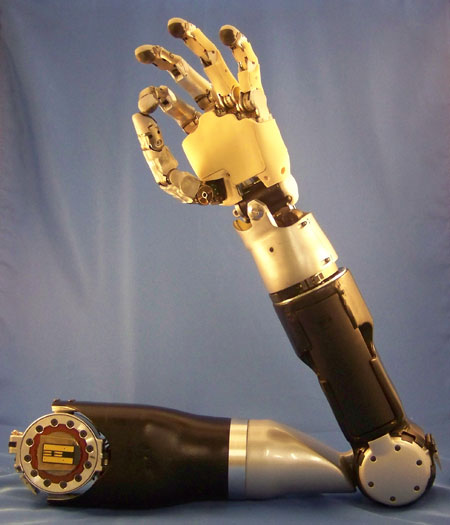The photograph features a detailed, machine-generated prosthetic arm designed with a robotic aesthetic. The arm, composed of various metallic and plastic parts, showcases a range of moving joints and components. The fingers of the hand are arranged to form an "okay" sign, with the thumb and forefinger creating a circle. The skeletal structure of the arm reveals yellow segments at the fingers with brown wires at the joints, and brown plastic sections in the forearm. A series of silver circular joints, peppered with dark-colored holes, connect different sections including the wrist, forearm, and upper arm. This intricate assembly is set against a muted blue cloth backdrop, which features wrinkles and provides a neutral setting that contrasts with the arm's metallic and plastic finishes. The backdrop covers both the floor and the wall, creating a cohesive background for this sophisticated prosthetic arm.